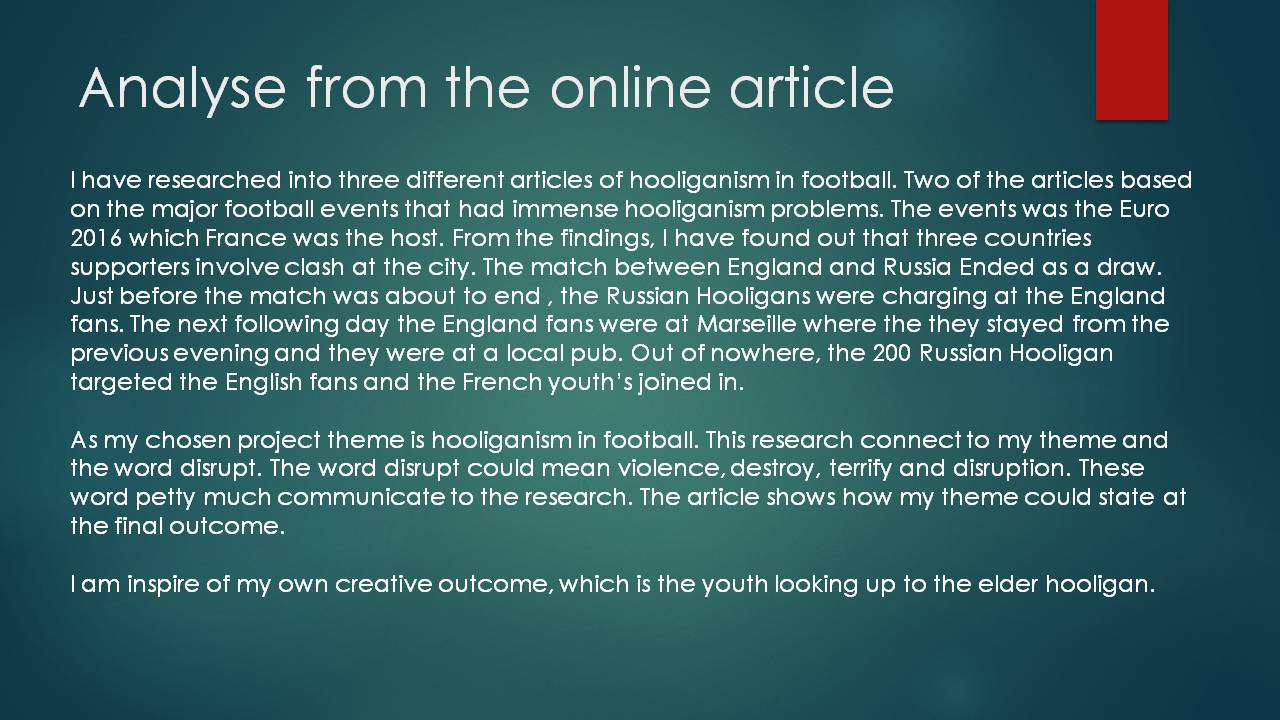The image is an excerpt titled "Analysis from the Online Article," displayed with white text on a dark green background, featuring a small red stripe in the top right corner. The text discusses research into three articles on football hooliganism, particularly focusing on two major events with significant problems: Euro 2016 hosted by France. It details clashes involving supporters from three countries, with specific emphasis on an incident where Russian hooligans charged at English fans just before the match between England and Russia ended in a draw. The following day, around 200 Russian hooligans, joined by French youths, targeted English fans at a local pub in Marseille. The presentation aims to reflect on hooliganism in football and its destructive impact, with a creative outcome of portraying youth influenced by elder hooligans, albeit with noticeable grammatical errors and a unique yet straightforward format.